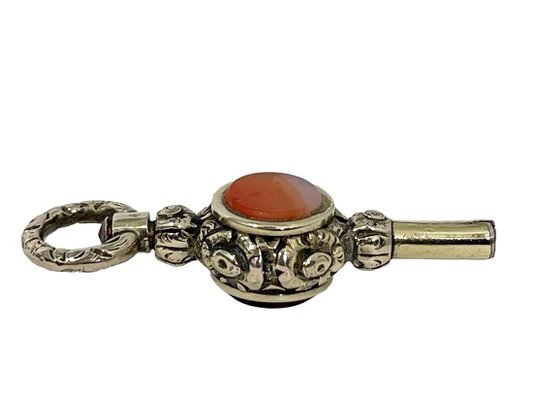The image depicts a single, ornate object resembling an antique key, set against a white background. The key displays a unique blend of silver and faint goldish-orange tones, possibly due to tarnishing or rusting. On the left side, there is a metal ring featuring slight cuts, large enough to potentially allow a finger through it, suggesting it could be used for turning the key. Attached to this ring is a slightly rounded segment that connects to a bulbous section adorned with intricate patterns. At the top of this section sits an inset red gemstone, adding a touch of elegance to the design. Extending to the right is a cylindrical extension, which might be intended for insertion into a keyhole to unlock something. The design and detailed craftsmanship make it reminiscent of a genie's lamp or other antique artifacts.